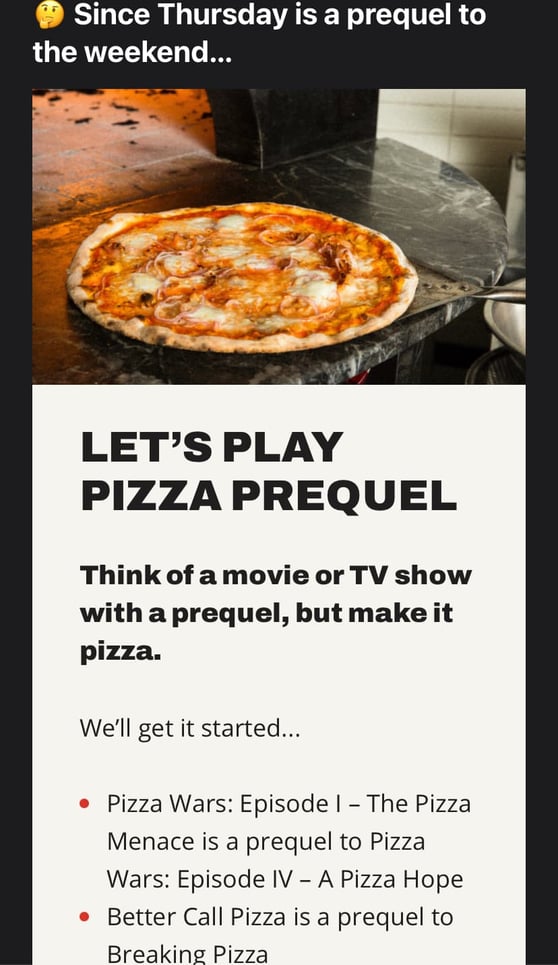This mobile screenshot lacks top indicators such as battery, Wi-Fi, or power status, surrounded by a black border that is thicker at the top. 

Centered in the upper black border is a thinking emoji followed by text in white font: "Since Thursday is a prequel to the weekend..." Below this is a small box displaying an image of a granite countertop with a cheesy pizza on it. The pizza appears to be a flatbread or thin-crust variety with visible mozzarella bubbles, placed in front of what looks like a pizza oven.

Beneath the pizza image is a white box extending beyond the bottom of the visible portion of the screen. The discernible black text reads: "Let's play Pizza Prequel! Think of a movie or TV show with a prequel but make it pizza. We'll get it started: 'Pizza Wars: Episode 1 - The Pizza Menace' is a prequel to 'Pizza Wars: Episode 4 - A Pizza Hope.' 'Better Call Pizza' as a prequel to 'Breaking Pizza.'"

This playful caption suggests a game related to inventing pizza-themed prequels for popular movies or TV shows, inspired by the cheesy pizza shown.